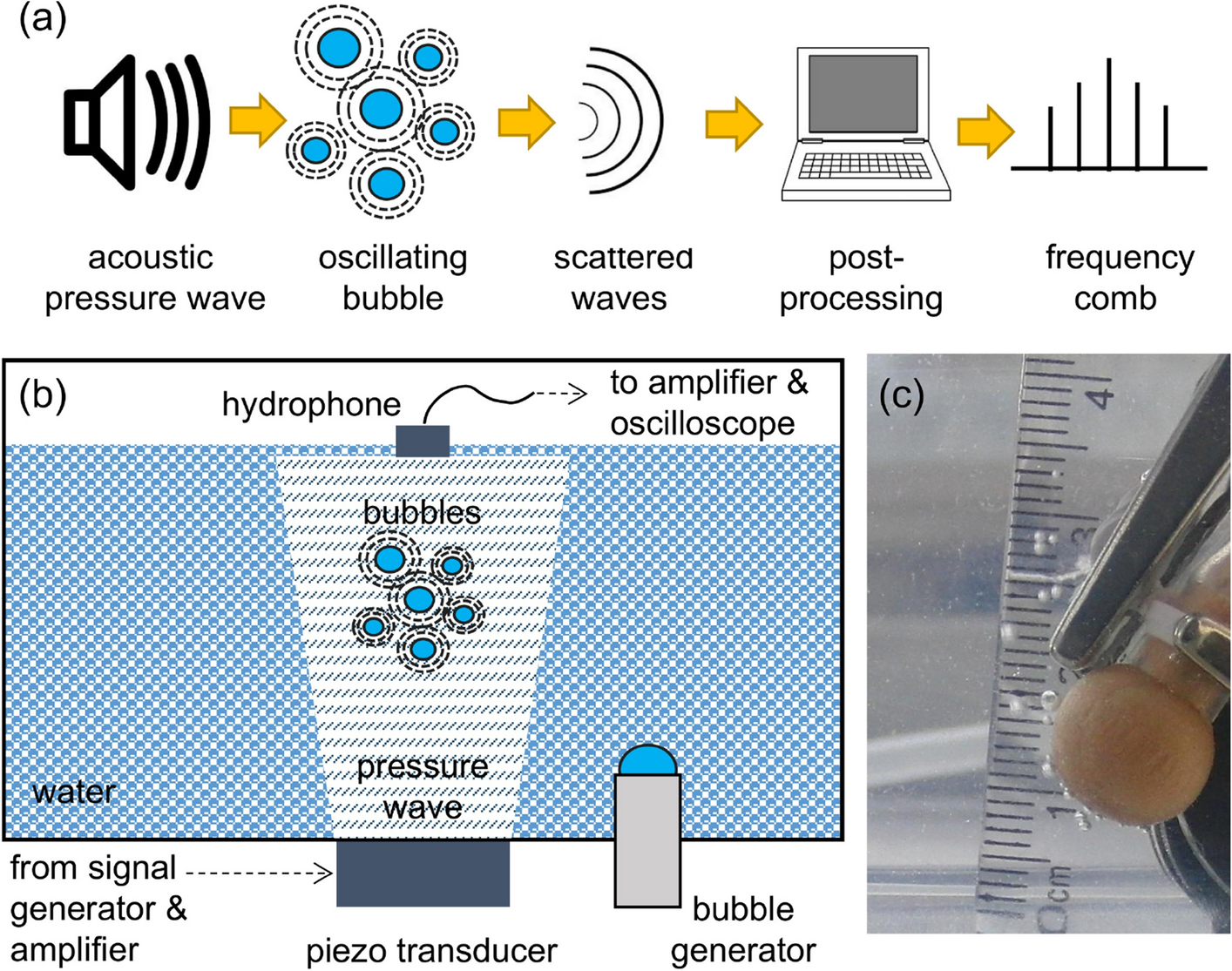This comprehensive illustration details a scientific process through a series of labeled images. At the top, an inset labeled (a) features a flowchart that begins with a speaker icon emitting sound waves, labeled "Acoustic Pressure Wave." A gold arrow directs attention to an area labeled "Oscillating Bubble," depicted by several bubbles. Another arrow points to four black semicircles, indicating "Scattered Waves," followed by another arrow leading to a laptop illustration with the label "Post Processing." The sequence concludes with a gold arrow pointing to a five-tiered loose pyramid of lines, labeled "Frequency Comb."

Below this flowchart is an illustration labeled (b). It shows a conical device submerged in water on a blue background marked with the word "Water" in the lower left-hand corner. Inside this device, "Pressure Wave" and bubbles are evident, connected to the words "To Amplifier and Oscilloscope" via a wire. This section also includes the device components: a "Hydrophone," "Piezo Transducer," and "Bubble Generator," each connected by arrows and lines depicting their interaction and signal flow.

Adjacent to this, labeled (c), is an inset showing a submerged clear ruler with visible centimeter markings, presumably depicting a real-life photograph of the experimental setup detailed in the previous sections. This intricate diagram elaborately illustrates the stages of an acoustic pressure experiment, detailing the transition from initial signal generation to final post-processing and frequency analysis.